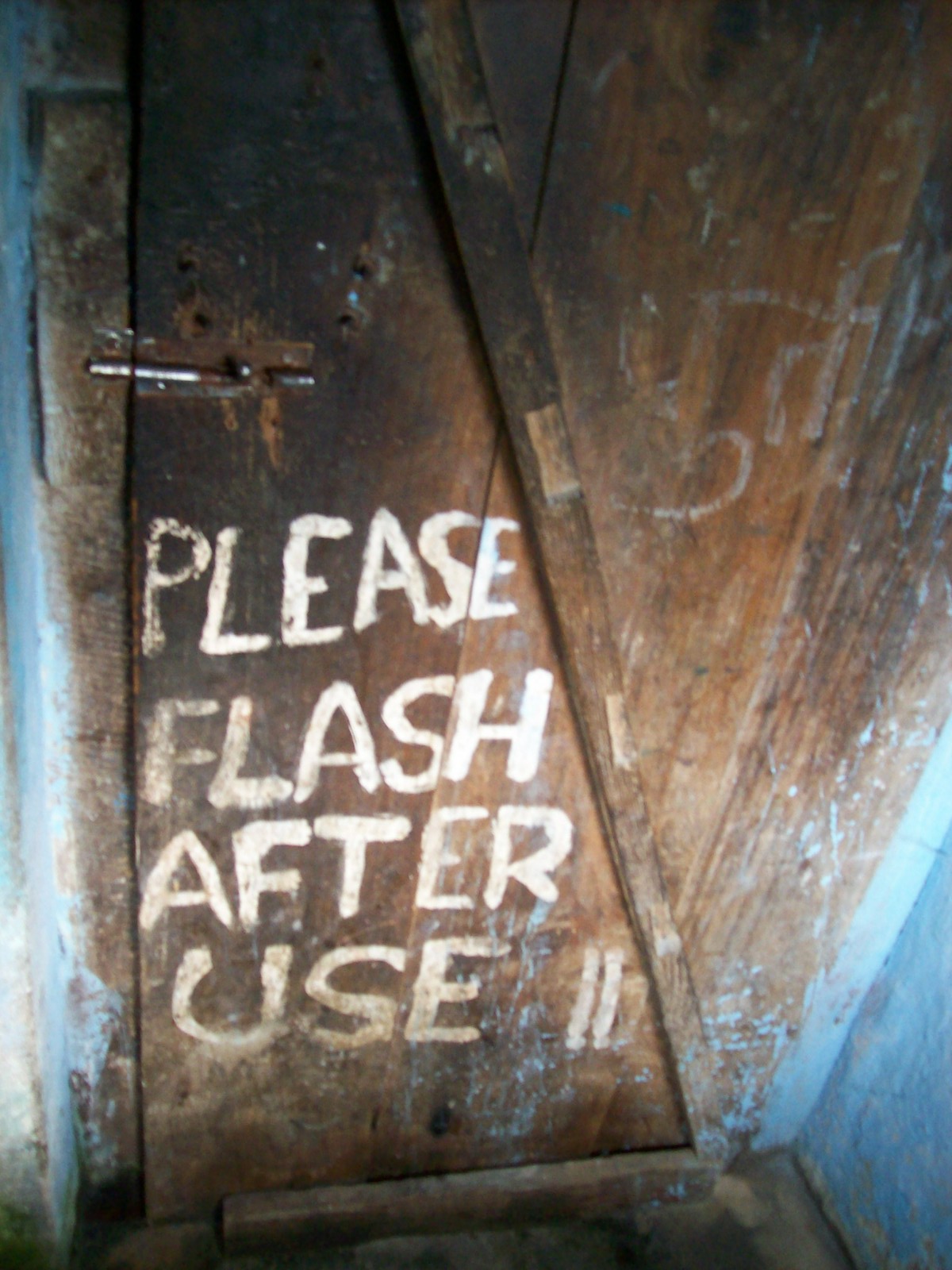The image depicts an aged and deteriorated wooden bathroom door, likely in a rustic cabin. The door is reinforced with a diagonal wooden support running from the lower right to the upper left and features numerous marks and holes, likely from previous locks. Written in white paint across the door are the words "PLEASE FLASH AFTER USE," a likely humorous misspelling of "flush." The door is secured with a simple, slightly rusted metal slide lock. The surrounding walls, painted in a chipped and patchy blue, suggest the overall dilapidated condition of the structure. The colors in the image primarily include shades of brown from the wood, white from the paint, blue from the walls, and some silver from the metal lock.